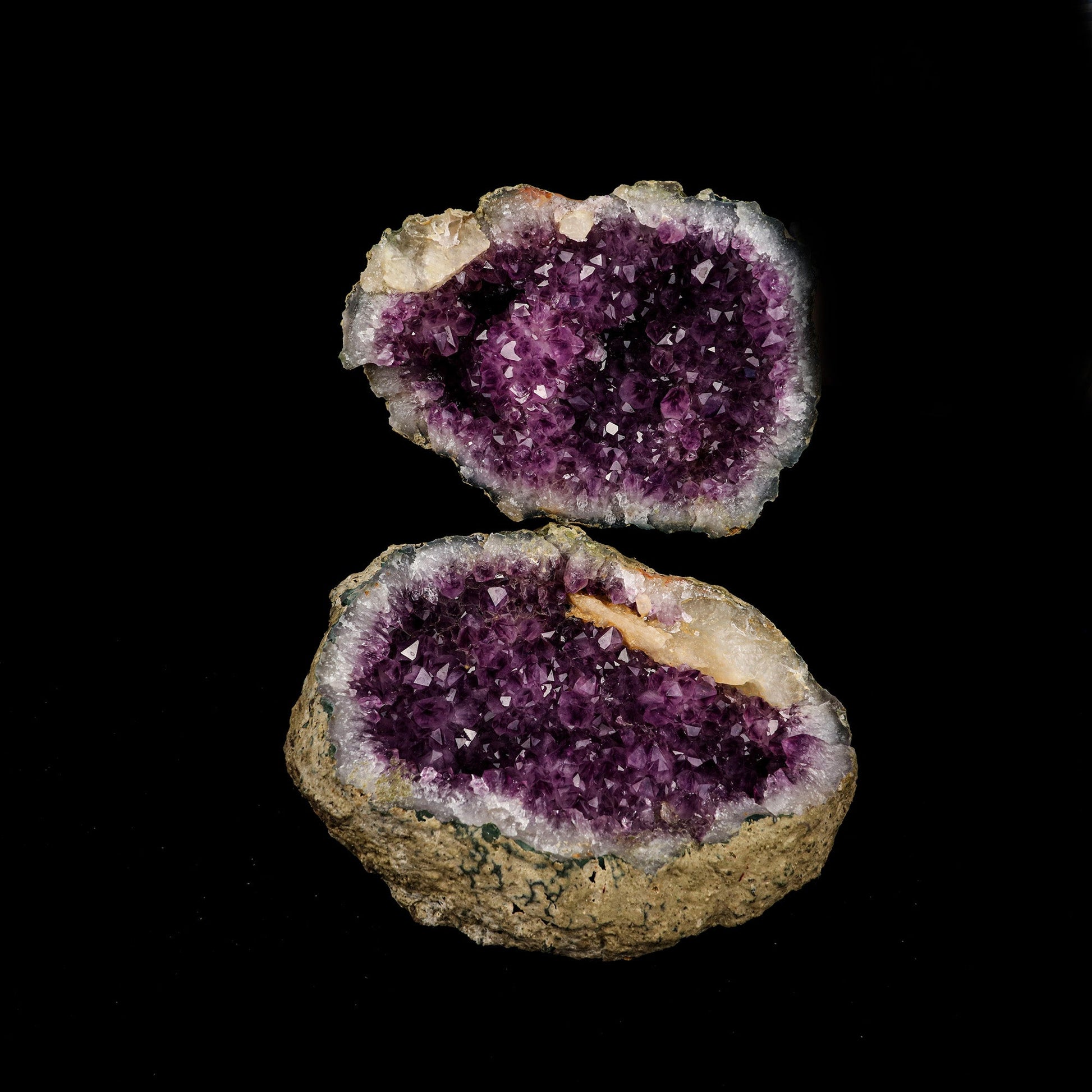This is a detailed photograph of a geode split into two halves, revealing its stunning interior. The exterior of the geode is a rough, pitted gray stone, somewhat resembling the texture of a coconut. The inner surfaces, once cracked open, display magnificent purple crystals surrounded by a ring of white, crystalline border. These highly reflective, many-faceted purple crystals shimmer under the lighting, giving an indication of the gemstone's potential high quality. The geode rests on a black background, possibly edited to enhance focus on the gemstone, with one half appearing to lean sideways. A hint of green and a slight tint of orange can be observed on the outer surface, adding more curiosity to its visual appeal. The photo, seemingly taken indoors under uniform overhead lighting, beautifully captures the intricate details and vibrant colors of this potential amethyst geode, suggesting that with proper polishing, it could become a stunning piece of jewelry.